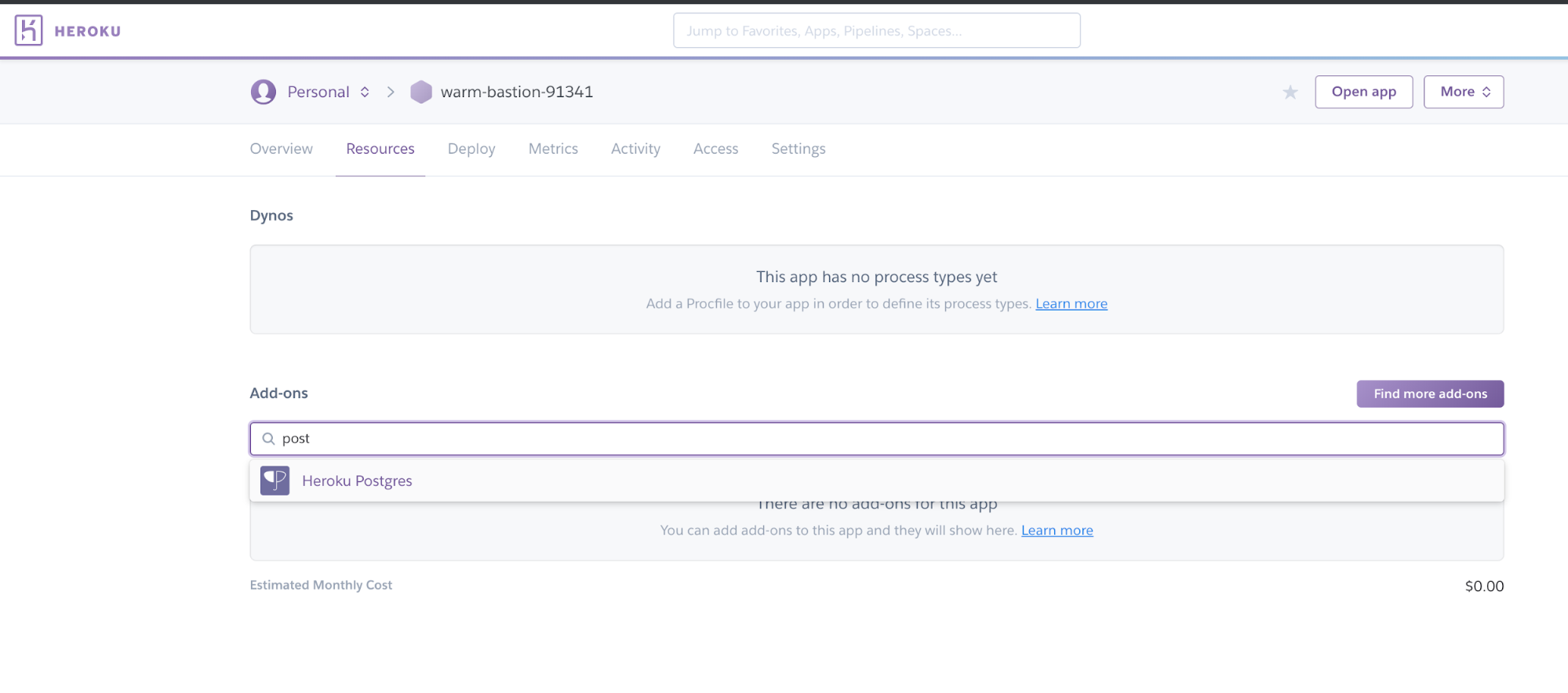The image depicts a Heroku interface with a white border at the top featuring the Heroku logo and an accompanying graphic design element to the left. On the right side of the top border, there is a search bar with text that is too small and blurry to discern.

Beneath the top border, there is a light gray section labeled "Personal," showcasing a generic profile picture icon along with a name and numbers that are too small to read clearly. To the right of this information, there are two buttons with text that is also too small to identify.

Below this section, there is a navigation bar with the options "Overview," "Resources," and "Activity," followed by additional text that is too blurry to read. Underneath this bar, there is a light gray box stating that "this app has no processes yet," with some smaller, unreadable text below, and a blue hyperlink that is too blurry to decipher.

Further down, a purple rectangular box contains text that is also too small to read, with additional unreadable text situated to the far left of this purple box.